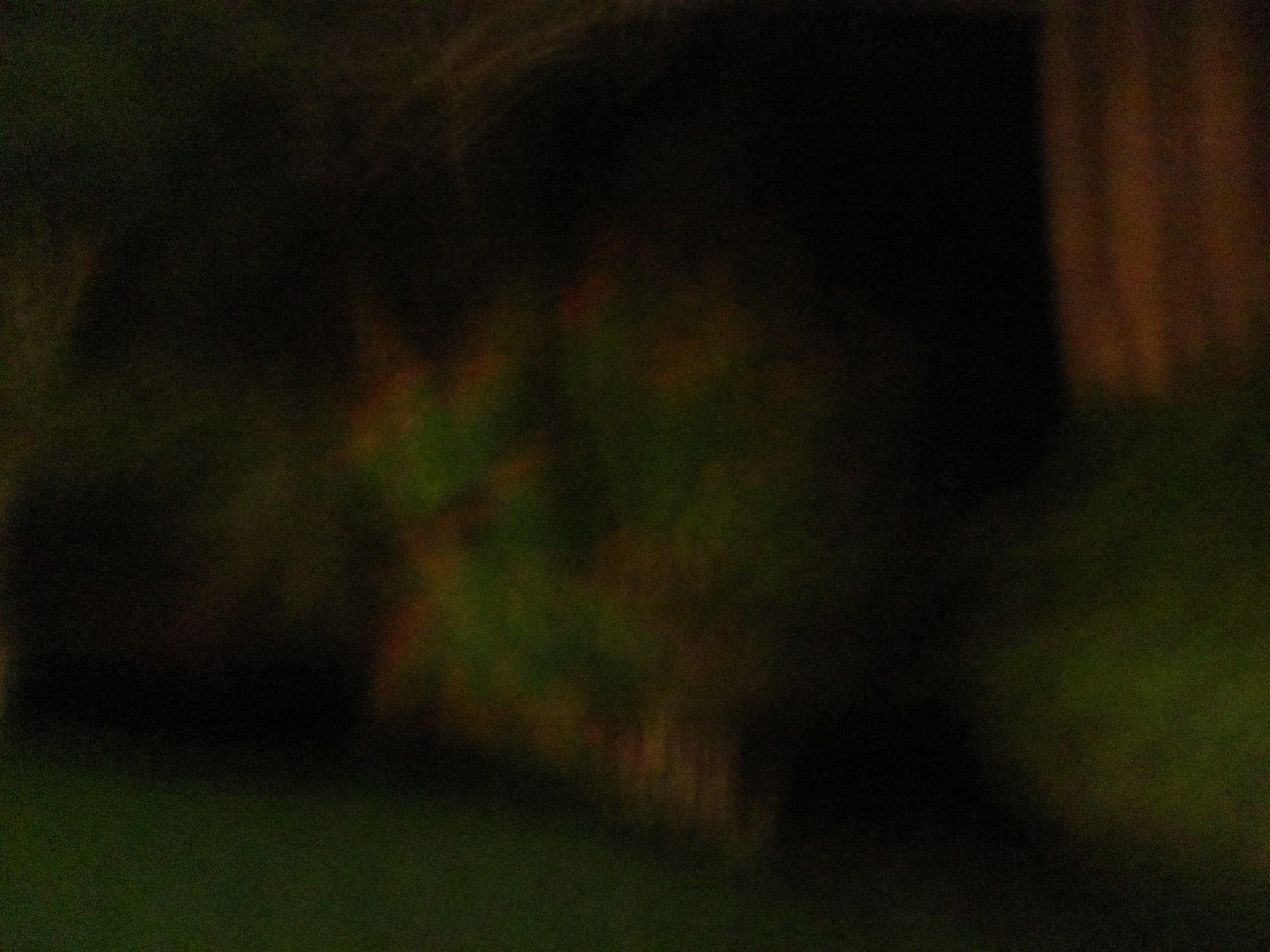This is a very dark, extremely blurry photograph, seemingly taken at night. The overall image is primarily black, with a few distinct color blurs. On the right side, there's an indistinct, pinkish blur that faintly resembles blinds inside a house, set against a black void. Below these suspected blinds, another greenish blur can be seen. The left part of the image contains the main focus, which is more of this greenish-pinkish blur, surrounded by an encroaching darkness. Towards the bottom left, the blackness gives way to a slight change in color to light gray due to the blurriness. The overall scene is extremely difficult to discern, but possible interpretations suggest it might depict a front yard with green bushes up against a house. However, the image quality is too low and indistinct to be certain about any specific objects.